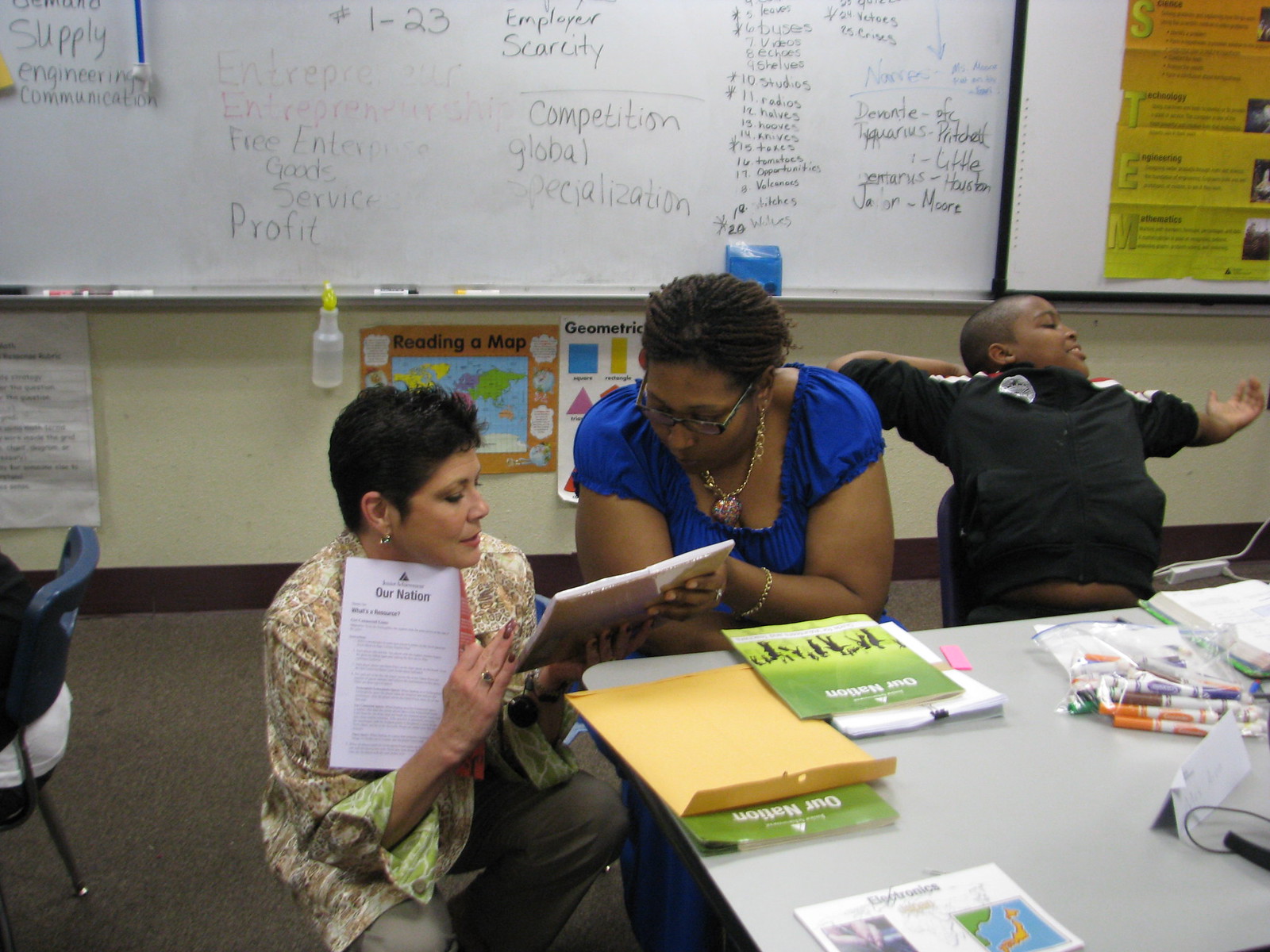In a lively classroom scene, a richly detailed background sets the stage with a whiteboard covered in extensive black writing and various educational posters, including ones labeled "Breathing and Math" and "Geometric". In the foreground to the right, a black boy in a black jacket stretches his arms backward, leaning against his chair, with a book and markers spread out on the table in front of him. To his left, a black woman with short black hair and wearing black glasses and a bright short-sleeved blue shirt is engrossed in a book, holding it with one hand while another woman, kneeling beside her, also holds the book. This second woman, dressed in a multicolored long-sleeved shirt, collaborates closely with the seated woman. Further on the table, various craft supplies, including markers, papers, and two green booklets titled "Our Nation," suggest the women are preparing or discussing educational content and possibly presenting it to the children, who appear to be engaged in a creative activity.